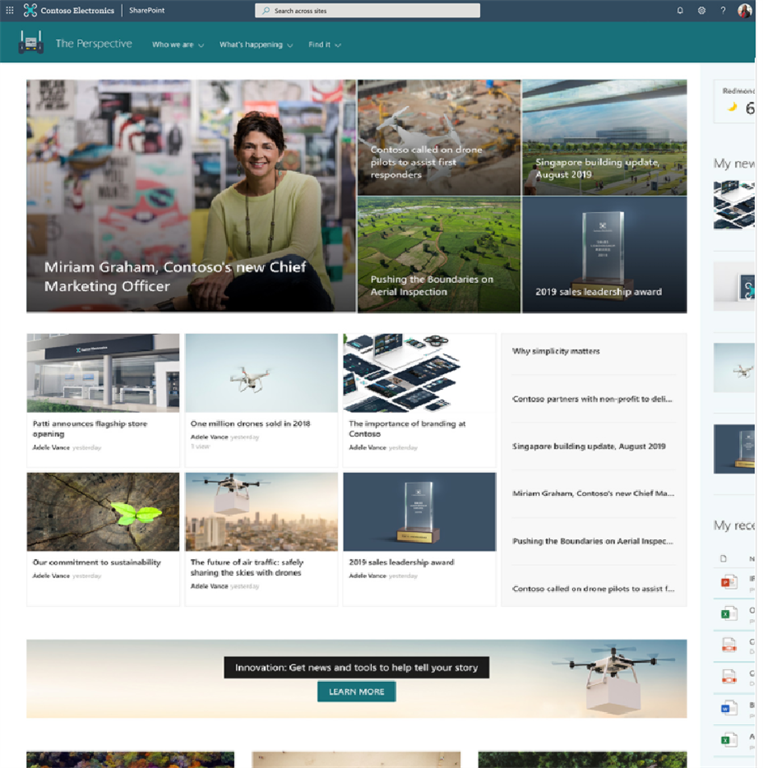A screen capture of a website’s homepage showcasing a comprehensive layout featuring navigational and visual elements. Centered at the top is a search bar, immediately followed by a horizontal menu bar for site navigation. The upper section of the page prominently displays a striking image of Miriam Graham, Consanto's new Chief Marketing Officer, seated in a blurred warehouse or store setting. This primary image is positioned on the left and is balanced by a set of four smaller, equally sized images on the right. These images provide aerial perspectives of grasslands, buildings, and construction sites, collectively occupying the same amount of space as the larger image.

Directly beneath these four images are six even smaller photographs, each with descriptive black text below, scattered evenly across the page to maintain visual harmony. The bottom portion of the webpage features a long rectangular image showcasing a drone, adding a technological flair to the overall composition. This well-organized layout effectively combines text and imagery to communicate the content clearly and engagingly.